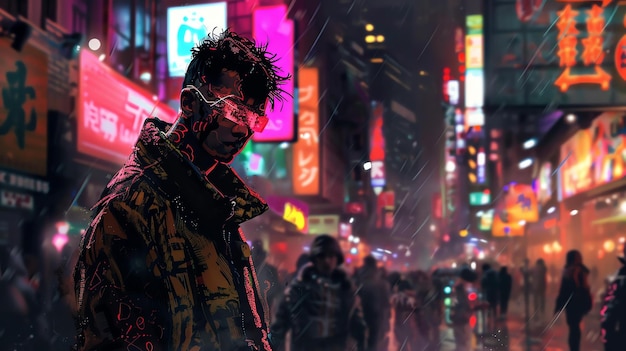This vibrant nighttime street shot captures a bustling urban scene in downtown Tokyo, Japan, characterized by towering buildings adorned with brightly lit neon advertisements in various colors such as hot pink, red, orange, green, white, and blue, all featuring Japanese text. The photograph is in landscape mode, showing a man standing prominently in the foreground. He has dark, very spiky hair and is donning futuristic, bright pink rectangular sunglasses. His attire includes a distinctive dark puffy winter coat with a large stand-up collar, emblazoned with a subtle brown satin detail. The reflection of the neon lights glistens on his neck and face, adding to the futuristic feel. To the right of him, in the softly focused background, other figures clad in dark clothing can be seen on the rain-slicked street, among them a man wearing a military uniform and helmet. The overall impression is one of a lively, modern metropolis alive with color, light, and movement.